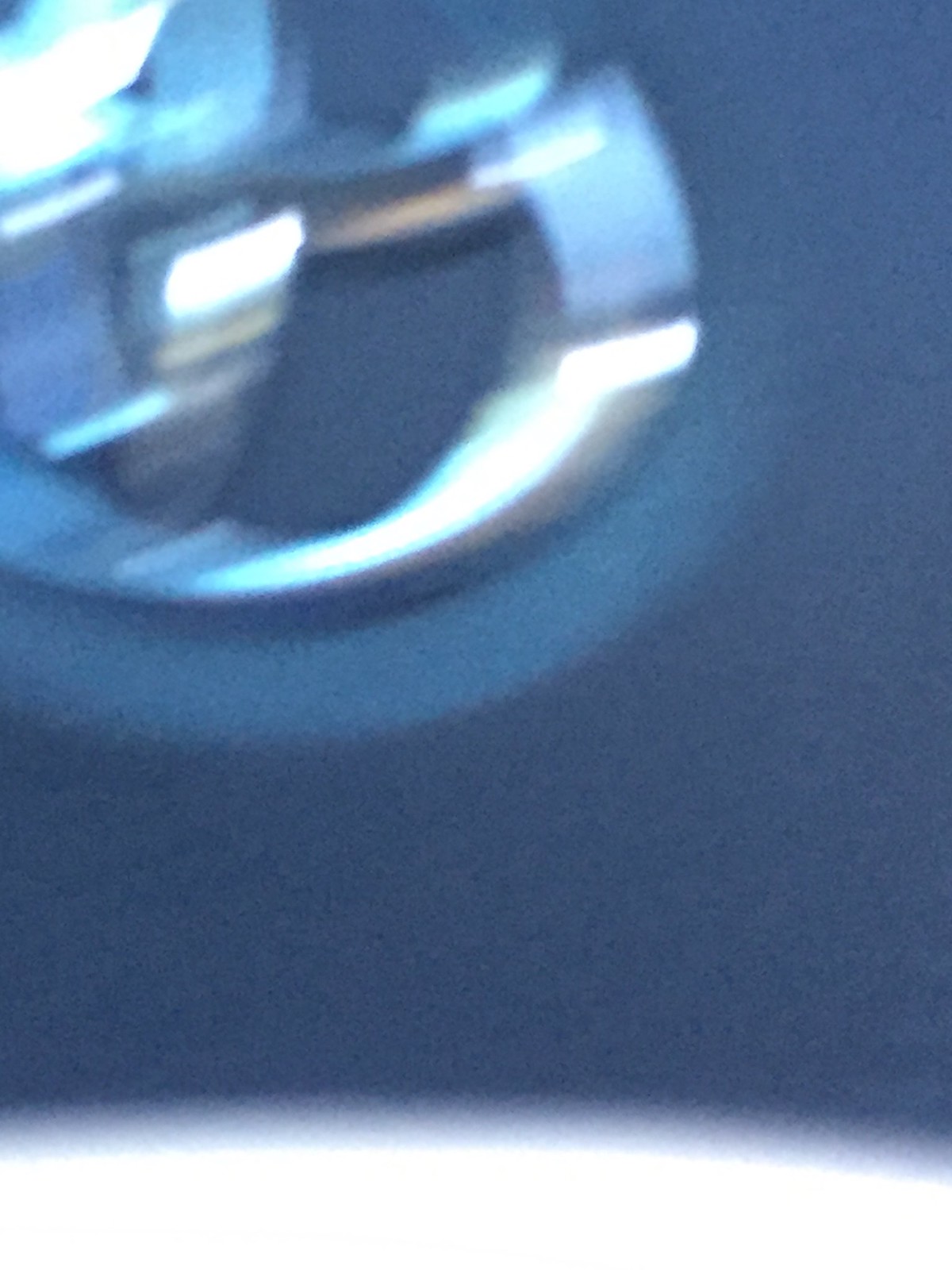A highly grainy and blurry photograph, potentially capturing a car's steering wheel. Dominating the center is a dark, grayish-black blob that likely represents the wheel itself, with a silver emblem embedded in the middle. The glare and reflections from the emblem contribute to the overall indistinctness, making it challenging to discern specific features. The light pollution around the emblem and the camera shake give the impression of an unstable shot, adding to the photograph's overall lack of clarity.